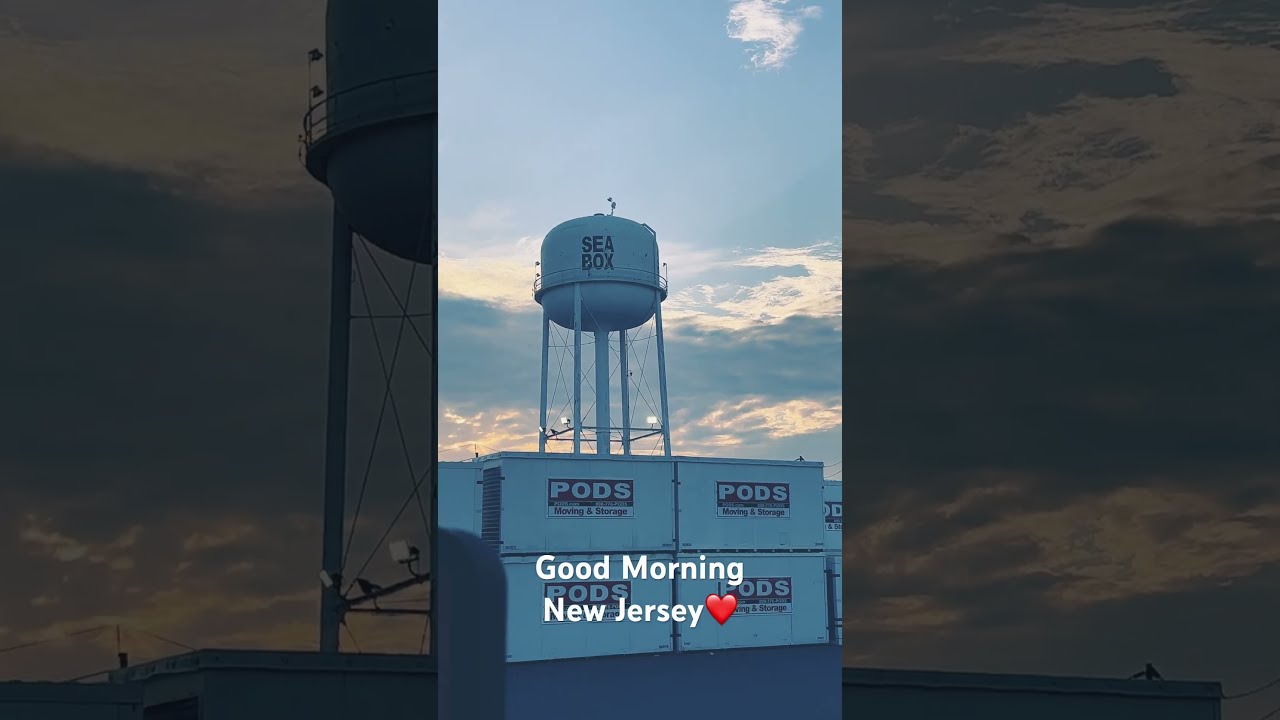The image is a photograph taken outside on a slightly cloudy morning. The scene is divided into three sections, with the central section being the primary focus while the left and right parts are darker. The bottom of the image is centered with four white storage pods stacked in a two-by-two formation, displaying the word "PODS" in white font inside red boxes. Rising behind these pods and slightly off-centered to the left is a light blue water tower featuring the barely readable text "Sea Box" in dark blue font. The background sky is a blend of blue and white clouds, suggesting it is a pleasant day. At the bottom of the image, the phrase "Good morning, New Jersey" is written in white font, accompanied by a red heart emoticon. The photograph appears to be a casual snapshot likely meant for sharing on social media platforms like Snapchat, capturing a serene morning scene.